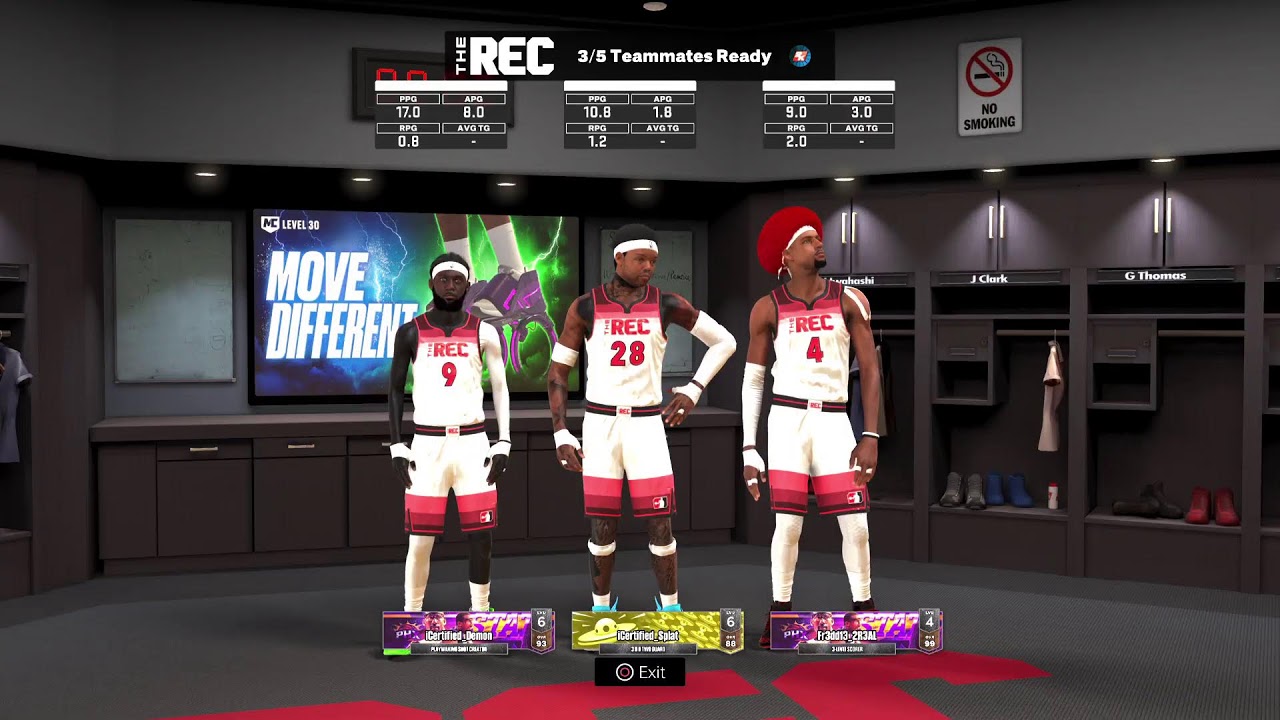This is a screen capture from what appears to be a mobile basketball video game, analyzing a recreation league match. The graphics are not highly detailed, indicating a possible mobile platform rather than a console. Displayed on the screen are three basketball players positioned centrally in a dimly-lit, gray-toned locker room. Each player dons a jersey that appears to be a hybrid of designs from NBA teams like the Miami Heat, Washington Wizards, and Portland Trail Blazers. The jerseys are predominantly white in the center with red accents on the edges, especially noticeable on the shoulders and the bottom of the shorts. 

The player on the right stands out with a vibrant red afro. Behind the players is a screen displaying a sneaker advertisement with the slogan "Move Different." Lockers are visible in the backdrop, with individual player attributes displayed above each athlete. The heading at the top of the screen reads "Three of Five Teammates," indicating that the image is part of a selection or team management interface within the game.